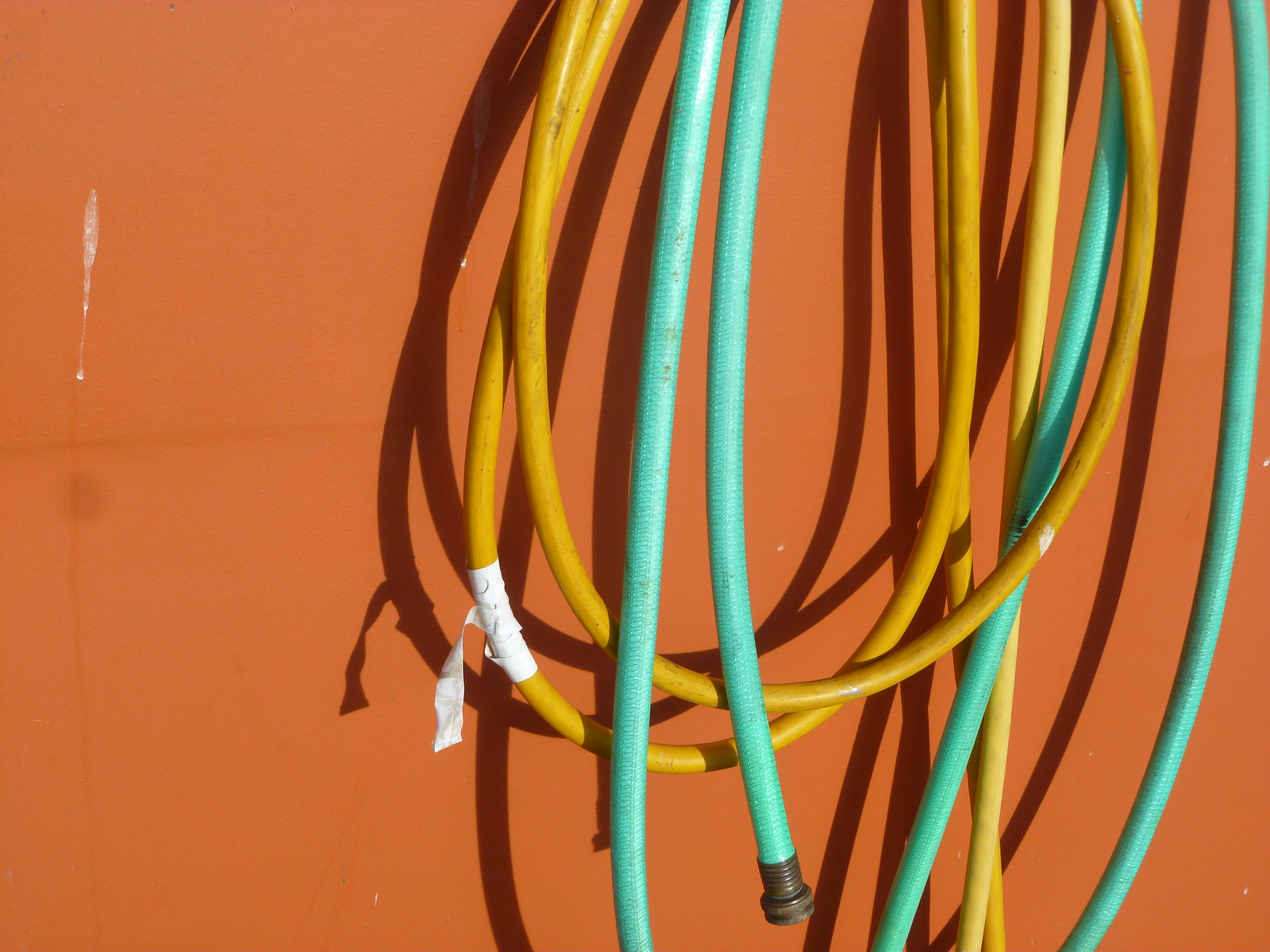The photograph depicts two garden water hoses, one light green and the other bright orange, neatly bundled and hanging from a structure in the top right-hand corner of the image. The orange hose is marked with white tape, possibly to prevent leaks, and both hoses show signs of use, with slight weathering. The hoses are wrapped around each other, creating a focal point that occupies the right two-thirds of the photo. Behind them, a dark reddish-orange wall can be seen, featuring drip stains and bird droppings in the top left-hand corner. The brass fittings of the hoses are visible at the ends, and the scene is brightly lit by sunlight, casting hard shadows of the hoses on the wall.